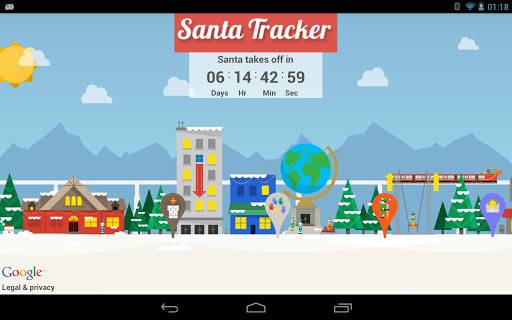The image is a screenshot from an Android device. In the top left corner, there is a small logo, while the top right corner displays the battery and Wi-Fi strength indicators. Dominating the main screen, the headline "Santa Tracker" is prominently presented in bold white text on a vibrant red background. Beneath this, a countdown clock with black text on a white background shows that Santa takes off in 6 days, 14 hours, 42 minutes, and 59 seconds. In the bottom left corner, the Google logo is visible. The backdrop of the image depicts a wintery city scene with snow-covered ground and trees. On the left side, there is a red building, and towards the center, a taller grey building and a smaller blue building can be seen. The background also features a range of snow-capped mountains, adding to the wintry ambiance.